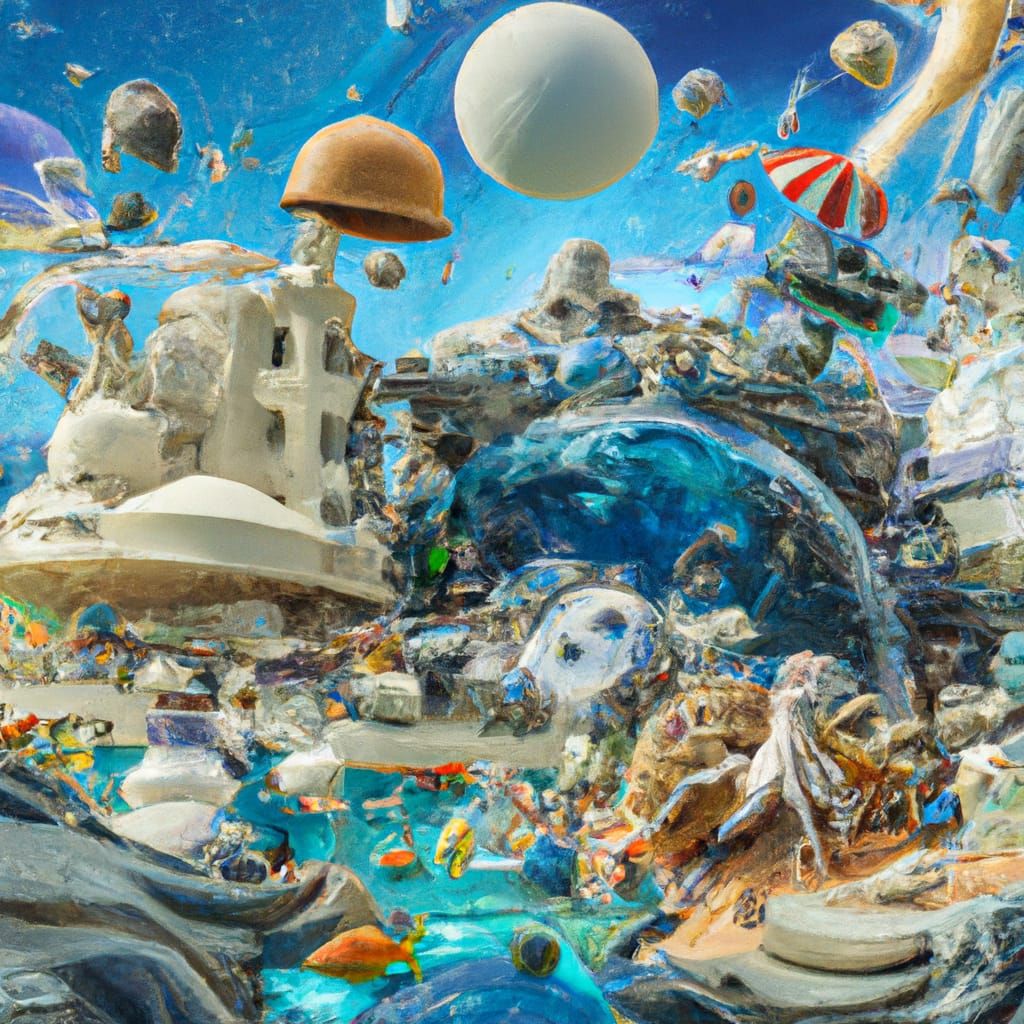This vibrant, vertically rectangular painting is a detailed collage depicting a bustling futuristic cityscape intertwined with an abundance of varied elements. Predominantly rendered in hues of blue, off-white, and grays, with sporadic bursts of color, the image is action-packed and visually engaging. At the bottom center lies a stretch of ocean, populated with fish, jellyfish, and rocks, enhancing the aquatic ambiance. Rising from the water are high-rise buildings and structures, suggesting a modern metropolis. The sky above is animated with floating objects such as red and white parachutes, colorful balloons, helmets, and even fish soaring amidst the clouds. Dominating the upper center is a large white ball, potentially a planet or moon, casting its glow over the busy sky. Additional elements like sails, an aquarium-like structure, and a sandcastle add to the eclectic mix of imagery. This intricate artwork, with its myriad life forms and objects, invites viewers to spend ample time discovering its numerous detailed components, making it a captivating piece that both intrigues and overwhelms with its complexity.